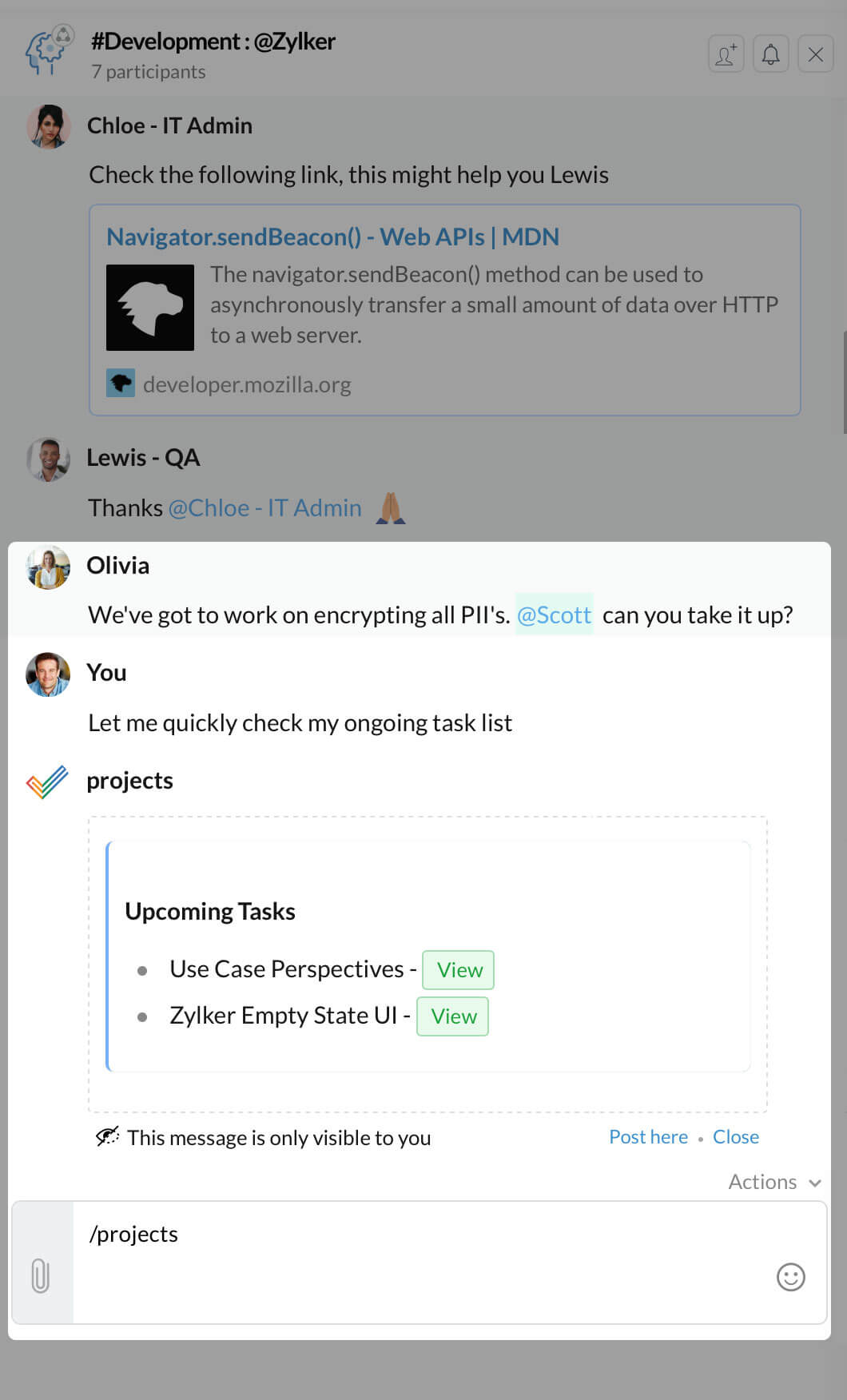This is a screenshot featuring several UI elements from a communication or project management platform. 

- In the upper left-hand corner, there is a light blue logo. 
- To the right of the logo is a bolded black text reading "#development:", followed by the handle "@zylker" in blue. 
- Below that handle, there is light gray text, although its content is not specified. 

Further down to the left, there's a profile picture:
- To the right of this picture, the small bolded black text reads "chloe-itadmin".
- Two lines down, there's another bolded black message: "Check the following link, this might help you Louis."

Below this message, a blue-outlined rectangle contains:
- A blue heading that reads "Navigator.sendBeacon Web APIs MDN".
- A logo (unspecified) and three lines of small black writing beneath the heading.

A few lines below this, another profile picture is present:
- To the right, the text reads "Louis-QA".
- Below this, Louis has written "Thanks."

Further down, another white rectangle appears:
- In its upper left-hand corner, there's a profile icon.
- To the right of this icon, the text reads "Olivia". 
- Olivia's comment says, "We've got to work on encrypting all PII's," and she tags "@Scott" with the question "Can you take it up?"

Below Olivia's comment:
- There is another profile icon and the text reads "You".
- Below "You," it says, "Let me quickly check my ongoing task list."

Under this, a checkmark icon is present next to the word "Project", which is followed by a box listing upcoming tasks:
- The first task listed is "Use case perspective" with a green "View" button to the right.
- The second line lists "ZYLKERMDQI".